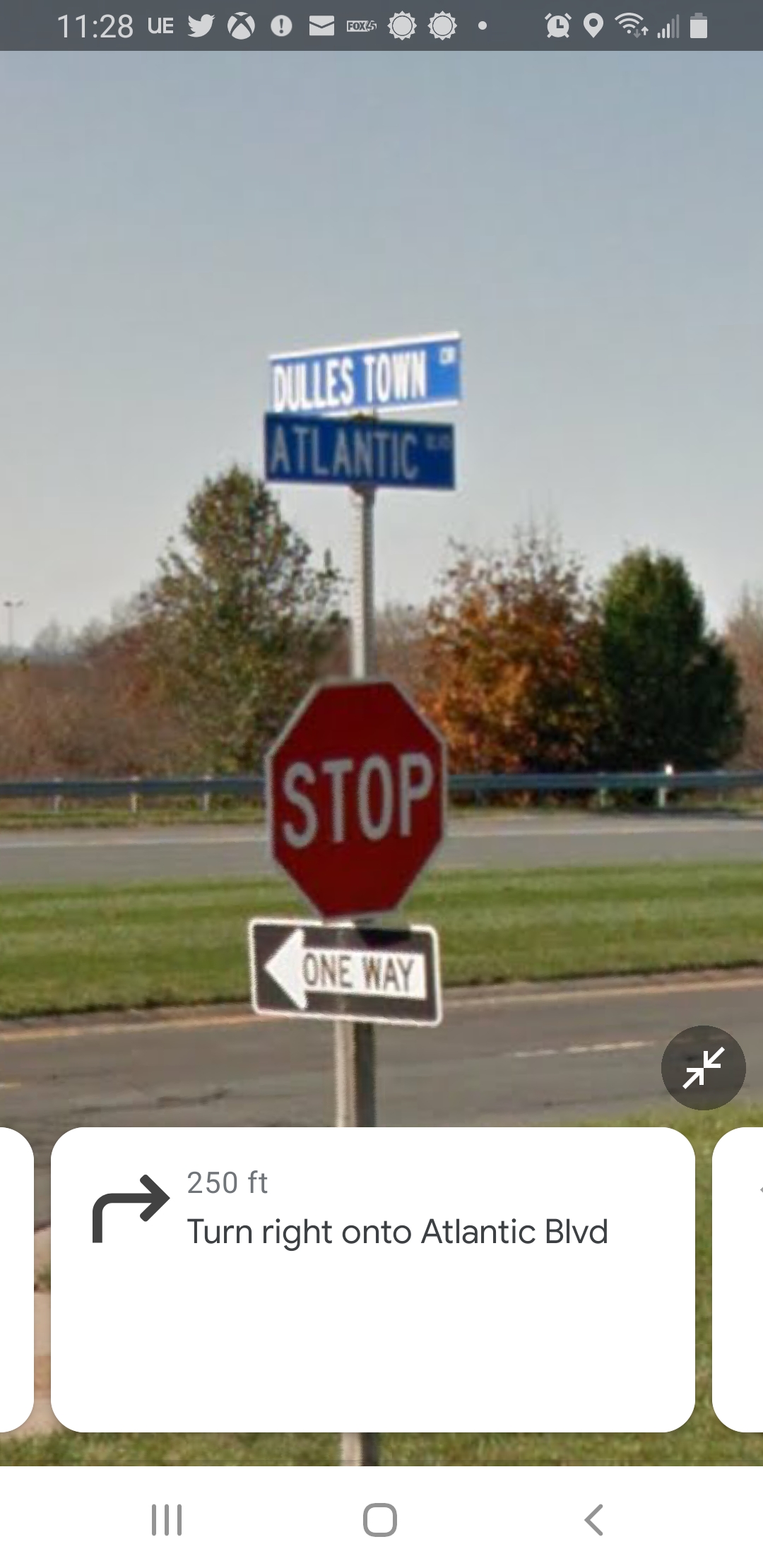This is a detailed screenshot of a smartphone displaying a navigation app, showing a live view of an intersection in a country setting under a grayish-blue sky. Prominently featured are several road signs mounted on a gray pole. At the top of the pole are two blue rectangular signs with white lettering; the upper sign reads "Dulles Town," while the lower sign indicates "Atlantic Boulevard." Beneath these, there's a red and white octagonal stop sign, and below it, a black and white "One Way" sign with a left-pointing arrow.

In the background, you can see patches of green grass and trees with varying foliage colors, predominantly green and some reddish-brown, suggesting a daylight scene without direct sunlight. On the opposite side of the road, there is another silver pole.

The screenshot includes a black border at the top with various smartphone status icons and information: "11:28," "UE," symbols for Twitter, Xbox, a round white circle with a black exclamation point, an envelope indicating a letter or email, two sun-like symbols, something that says "Fox," an alarm clock, a map pin, Wi-Fi, and a battery indicator.

At the bottom of the screen, there is a white rectangle with black lettering and a black right-pointing arrow, providing turn-by-turn instructions: "In 250 FT, turn right onto Atlantic Blvd." This suggests the image is from a mapping application, presenting real-time directions for navigating the intersection.